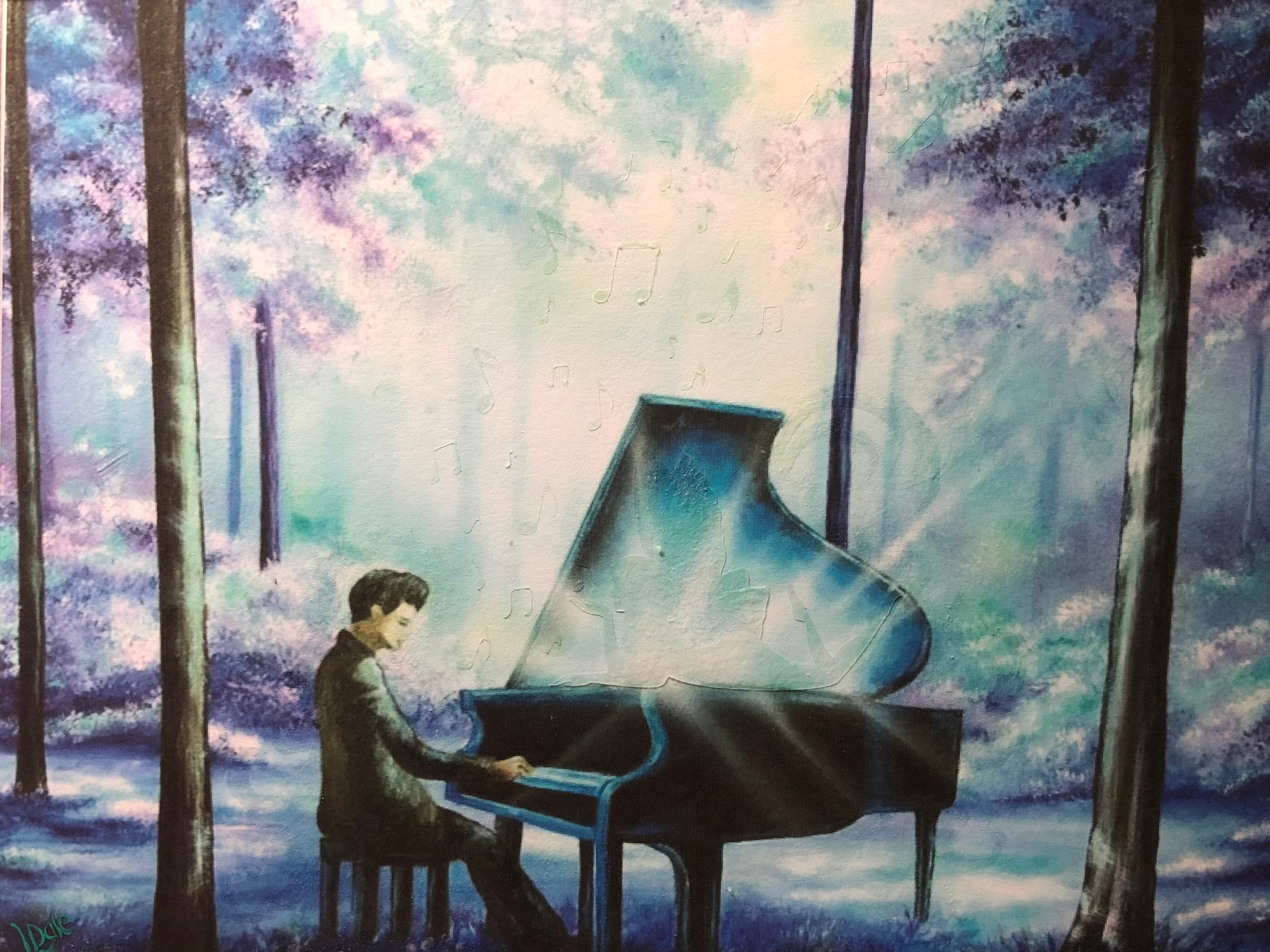This enchanting painting captures a serene young man playing a radiant black piano in a mystical forest. His dark brown hair frames a face engrossed in concentration, while he dons a green jacket and dark trousers. The piano's lid is open, emanating a bright white light, casting a glow on the surroundings. The backdrop is a forest clearing burst with vibrant colors—trees adorned with lavender, purple, and blue leaves amidst blue, teal, and green bushes. Light streams ethereally from above, adding to the otherworldly atmosphere. Subtly hidden among the foliage are small music notes drifting up from the piano, a testament to the artist’s meticulous attention to detail. This painting beautifully converges nature and music in a compelling, luminous scene.